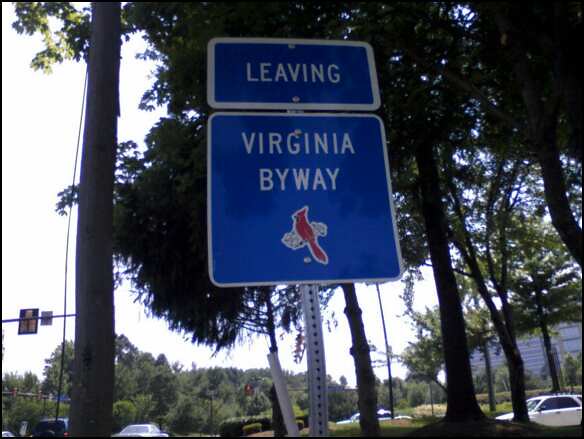The image depicts two road signs positioned vertically, one above the other, situated on the side of a road with a broad median strip filled with lush green grass and mature trees with slender, dark trunks and vibrant green foliage. To the left of the signs stands a tall telephone pole, which appears to be constructed from a white metallic material. In the background, additional trees and a variety of cars, including a notable white vehicle on the right, are visible. 

Both signs share a blue background with a white border and rounded edges. The upper sign, which is shorter, reads "Leaving" in white text. The larger, lower sign includes the words "Virginia Byway" in white, accompanied by an illustration of a red cardinal outlined in white.